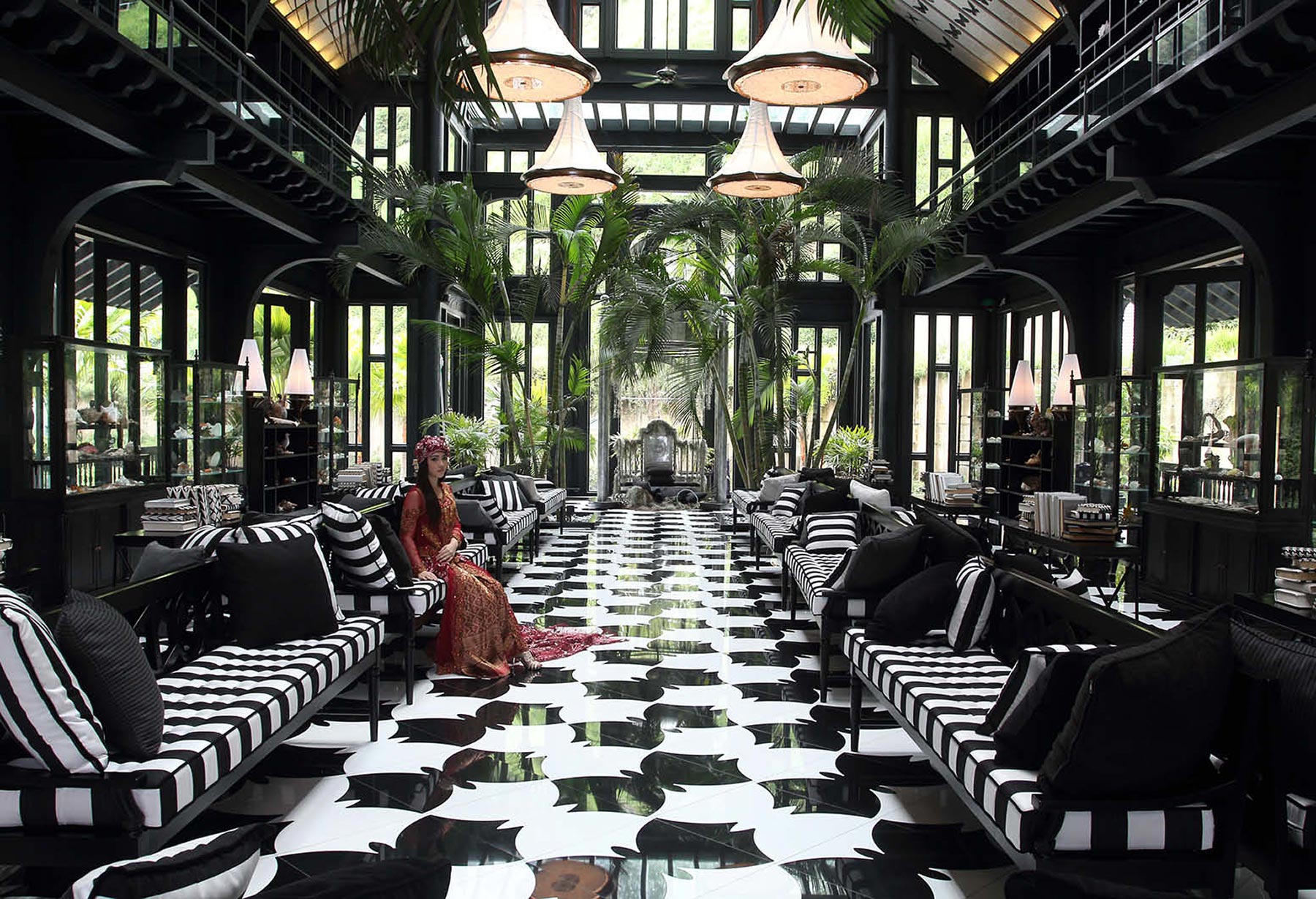The image showcases the interior of a luxurious and intricately designed sunroom, likely within a mansion. The room is elongated and features a striking black and white color scheme, with black and white striped couches flanking both sides. Each couch is adorned with matching black and white striped pillows. The floor is a glossy, smooth expanse of black and white tiles arranged in an elegant, butterfly-like design. 

Bringing a touch of nature indoors, the room is dotted with small, tropical-looking trees, including some palm-like varieties, contributing to the lavish ambiance. Along the left side, a series of black china cabinets with glass fronts display fine china and various items, while bookshelves can also be seen.

The sunroom is bathed in natural light that streams in from the numerous windows lining the walls and ceiling, complemented by four large lamps hanging from above. At the far end, an open doorway is flanked by additional greenery, enhancing the bright, airy atmosphere.

A woman dressed in a fancy, long-sleeved red and gold dress with a red hat and long brown hair is seated on one of the center-left couches. She adds a focal point of elegance to the room, her attire further accentuating the sophisticated setting.